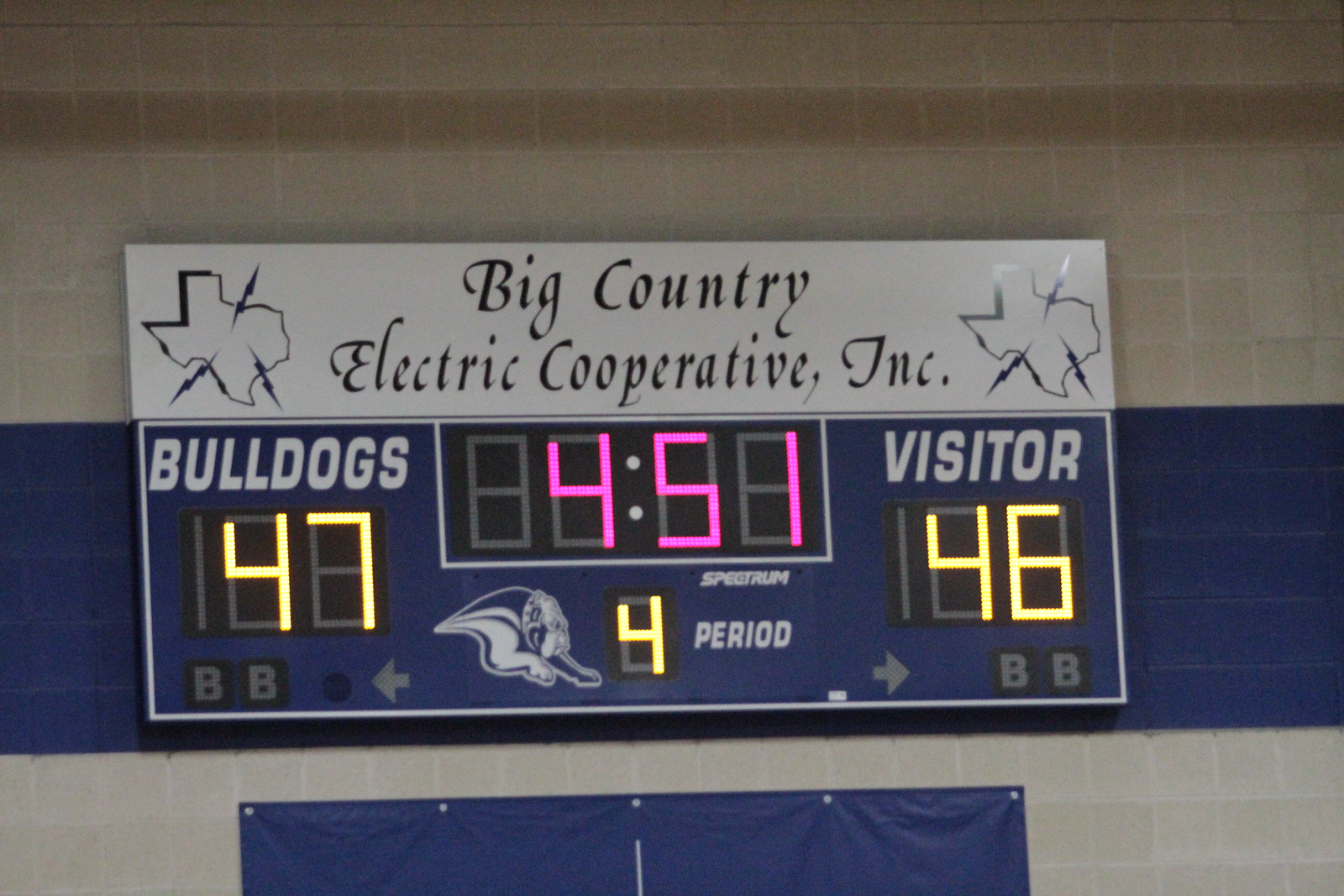This is a photograph of a blue scoreboard, prominently displaying the details of a basketball game. At the top, a white banner reads "Big Country Electric Cooperative, Inc." flanked by outlines of the state of Texas with lightning bolts running through them. The scoreboard shows the home team, the Bulldogs, leading with 47 points, while the visiting team has 46 points. It is the fourth quarter, with 4 minutes and 51 seconds remaining. The period indicator, positioned near a logo of a bulldog, shows "4". The scores and period are illuminated in yellow lights, while the time is shown in red lights. The scoreboard is mounted on a gym wall, which is white with a blue stripe, and below it hangs a blue tarp. This detailed setup emphasizes the competitive atmosphere of the game.